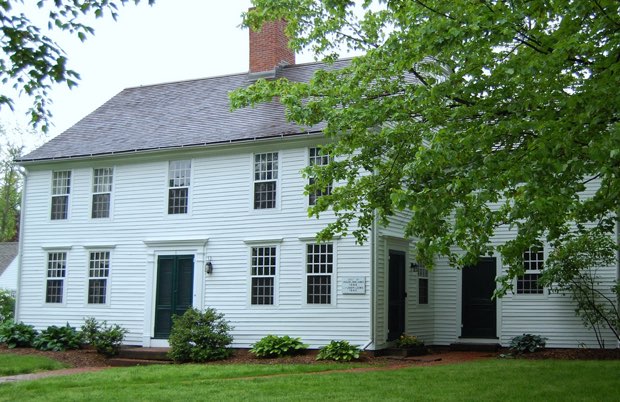The image depicts a large, two-story white clapboard-sided house with numerous windows. It features distinct architectural details, including a gray roof and a brick-red chimney. The main entry, located on the leftmost side, consists of dark gray double doors with Federalist ornamentation and brown steps leading up to a small stoop. Additionally, there are two more exterior doors: one black door on the rightmost wing and a side door on the main wing. In the foreground, a green lawn is accompanied by a red path, shrubs, and various plants. Branches from trees with dark and light green foliage frame the top corners of the image. The scene is set outdoors during the day, with a gray sky and another building slightly visible in the background.